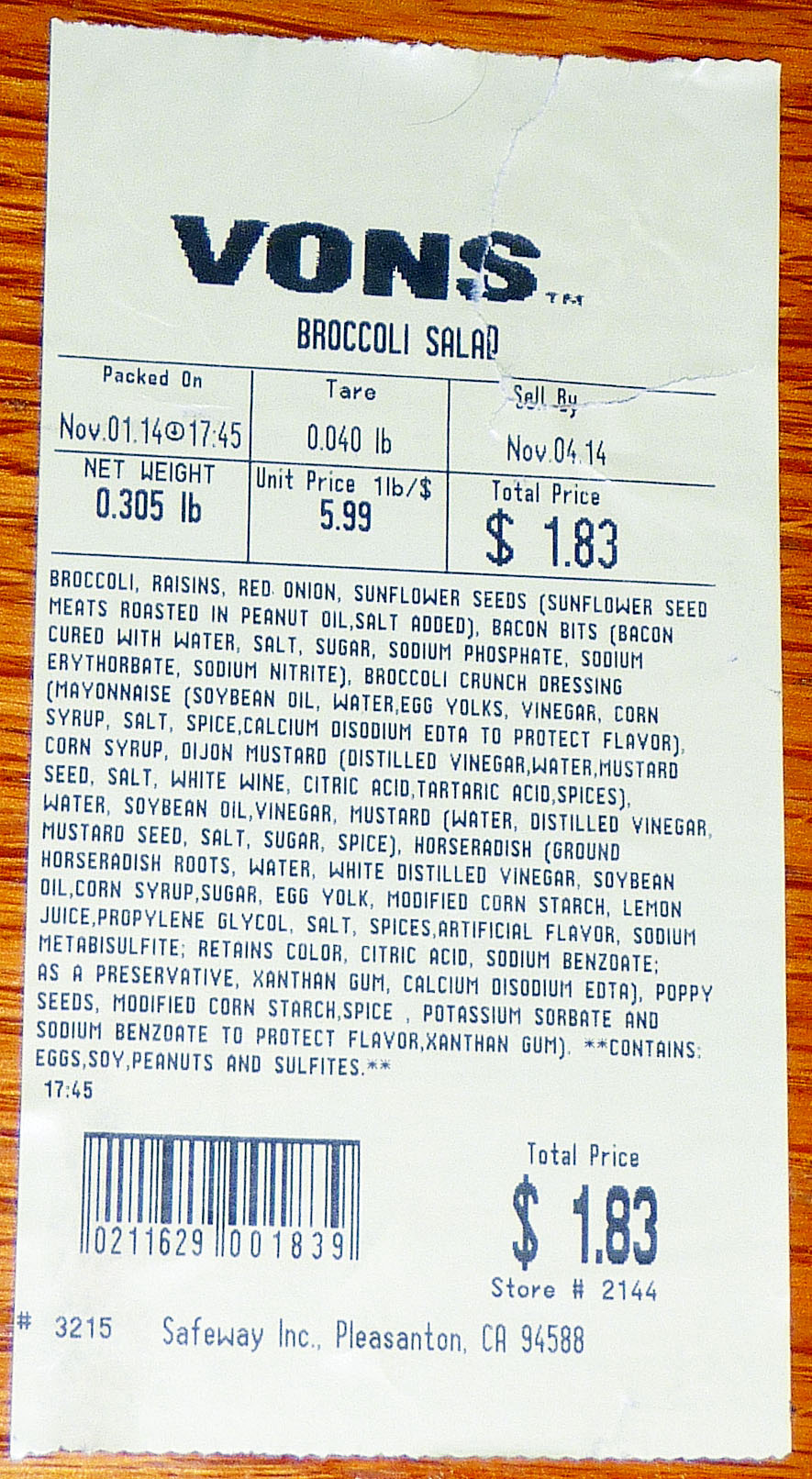The image features a white rectangular receipt from Vons grocery store, displayed on a brown wooden surface with a slight tear at the upper edge. The receipt is printed in black ink and prominently features "VONS" in bold lettering at the top. Below it, it identifies the product as "Broccoli Salad," detailed with several key pieces of information. The salad was packed on November 1, 2014, at 17:45 with a net weight of 0.305 pounds and a tare weight of 0.040 pounds. The unit price is listed as $5.99 per pound, resulting in a total price of $1.83. The receipt also includes a "Sell by" date of November 4, 2014. At the bottom, there is a barcode on the lower left and the store number 2144 on the lower right, alongside the repeated total price of $1.83. Additionally, the receipt notes "Number 3215 Safeway Incorporated, Pleasanton, California 94588." Information about the broccoli salad’s ingredients is also noted beneath the pricing details.